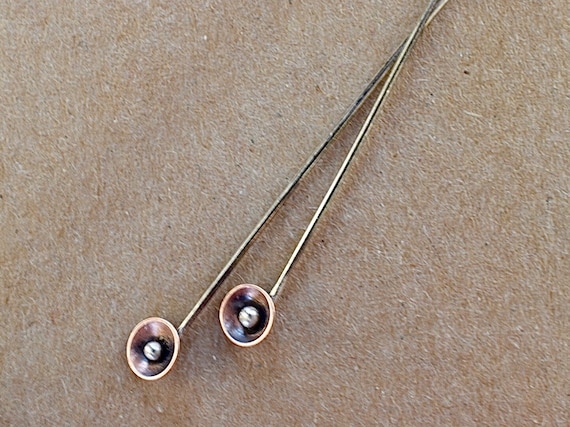The photo depicts a pair of interwoven objects with an ambiguous nature, resting on what appears to be a background that resembles skin or a fur-like material with black and white specks. The items are crisscrossed at the top, closely resembling ladies' hairpins or old-fashioned earphones but also bringing to mind stylized jewelry. Each piece terminates in a spherical end, described as either a round, stylized ball that could be made of mother-of-pearl, onyx, opal, or possibly a combination, potentially even featuring a suspended pearl or silver metal ball. The handles are metallic, lacking any modern comfort features like rubber, and suggest antiquity. The overall appearance shares similarities with devices used to extinguish candles, characterized by upside-down bell shapes that have hollow interiors and are accented by silver detailing.